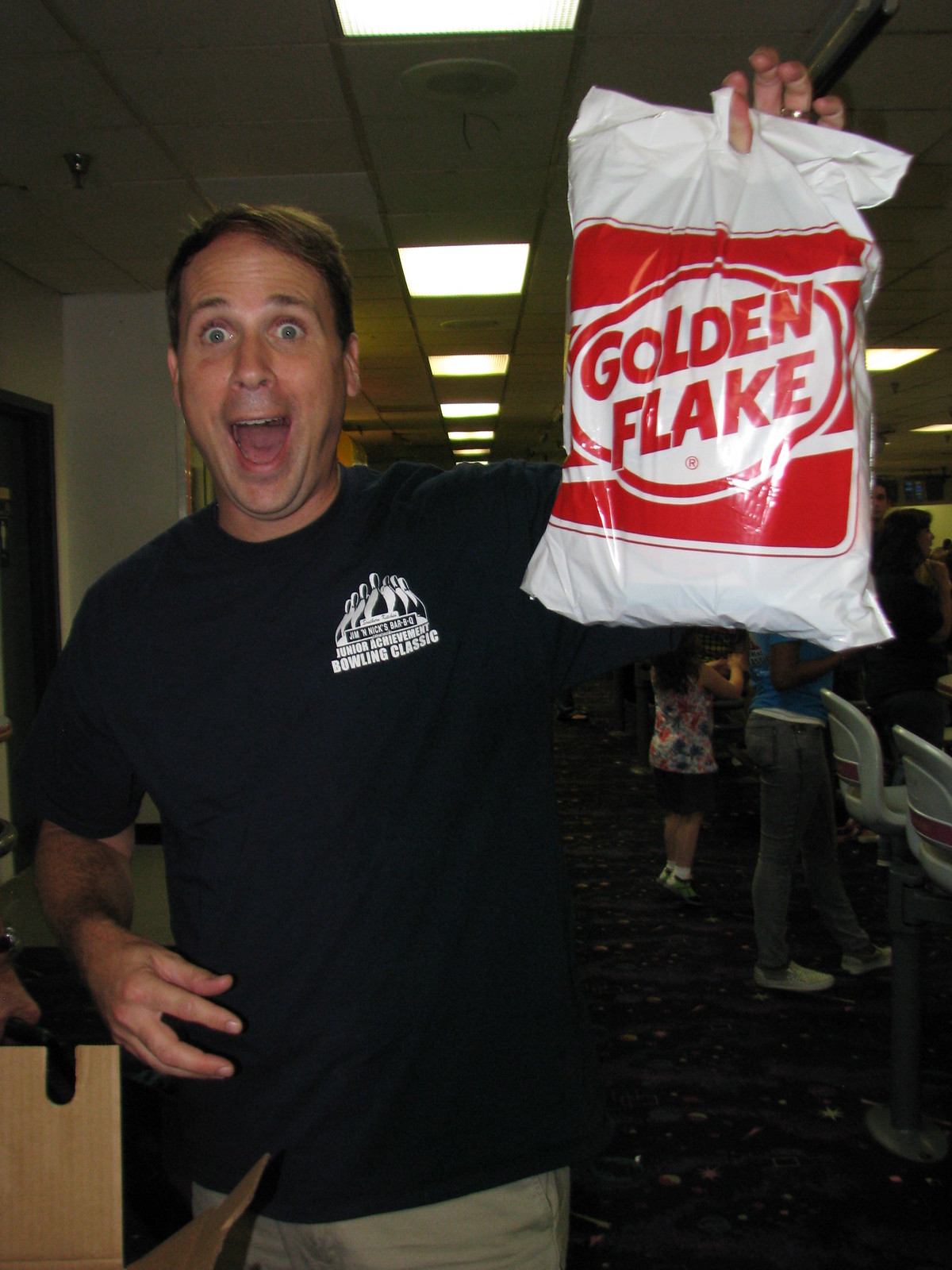The image depicts a Caucasian man, likely in his mid-30s to early 40s, with short brown hair, appearing on the left-hand side of the frame from the waist up. He has an exaggerated look of surprise or amazement on his face. The man is wearing a black, short-sleeved t-shirt with a white logo on the left side that reads "Junior Achievement Bowling Classic" and features bowling pins. He is holding up a large white chip bag labeled "Golden Flake" in his left hand. The bag's design includes a red logo consisting of a red circle with three horizontal stripes in the background, and the words "GOLDEN FLAKE" in capital red letters within the circle. The setting appears to be an indoor space, possibly an office or a facility, with some gray chairs visible on the right-hand side. The overall lighting of the image is dim but clear.